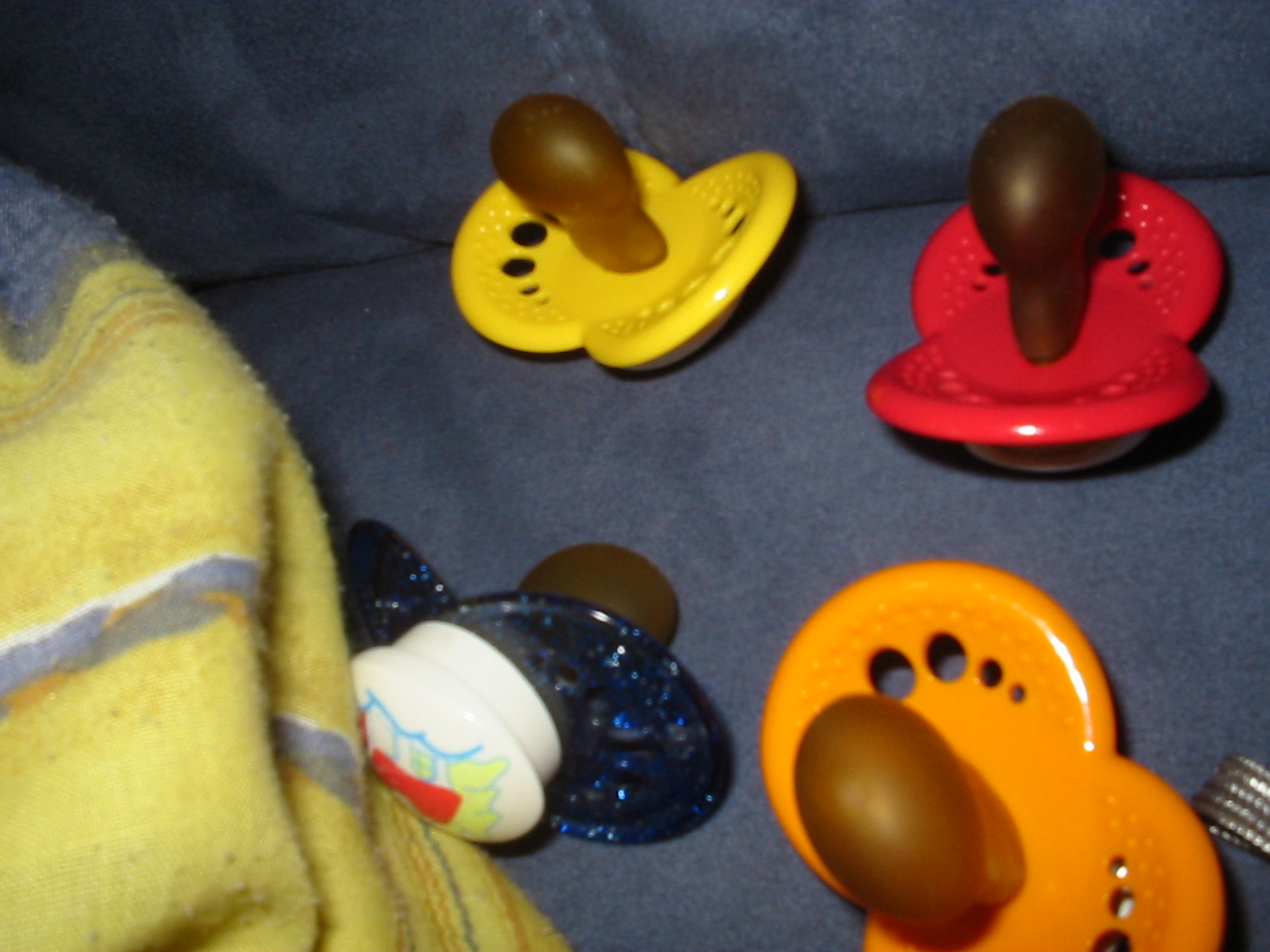This color photograph, although slightly blurry, captures a scene featuring four brightly colored pacifiers scattered on a piece of blue fabric which seems to resemble a seat or couch. The fabric extends upwards in the background, possibly suggesting the backrest of a couch or somebody's legs clothed in blue jeans. 

In the bottom left of the image, a child's blanket with yellow and gray stripes is visible. The pacifiers are arranged as follows: the top left pacifier is yellow with an orangish rubber teat. To its right, there's a red pacifier featuring a nearly brown rubber teat. Coming down next to the blanket on the left side, there's a blue glittery pacifier with a white back adorned with a picture, and it also has a brown teat positioned downwards. To the far right, there's another red pacifier with a brown rubber teat. 

Additionally, a small metallic object is barely visible in the extreme right-hand corner. The overall composition suggests a cozy, child-friendly environment filled with colorful and well-loved items.